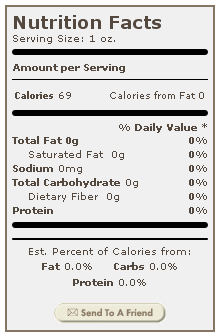This image showcases a vertical, portrait-oriented Nutrition Facts label set against a white background with a black or gray pixel border. The label is divided into several sections. At the top, in prominent letters, it reads "Nutrition Facts". Below this, it specifies "Serving Size: 1 ounce" and "Amount Per Serving: Calories 69, Calories from Fat 0". A deep black line segments the next part, listing the nutrient content: Total Fat 0 grams, Saturated Fat 0 grams, Sodium 0 milligrams, Total Carbohydrate 0 grams, and Dietary Fiber 0 grams, with all values reflected as 0% in the Percent Daily Value column on the right. Another black line follows before stating the "Estimated Percent of Calories from Fat 0.0%, Carbs 0.0%, Protein 0.0%". At the very bottom, a feature is shown with an accompanying envelope icon stating, "Send to a Friend".